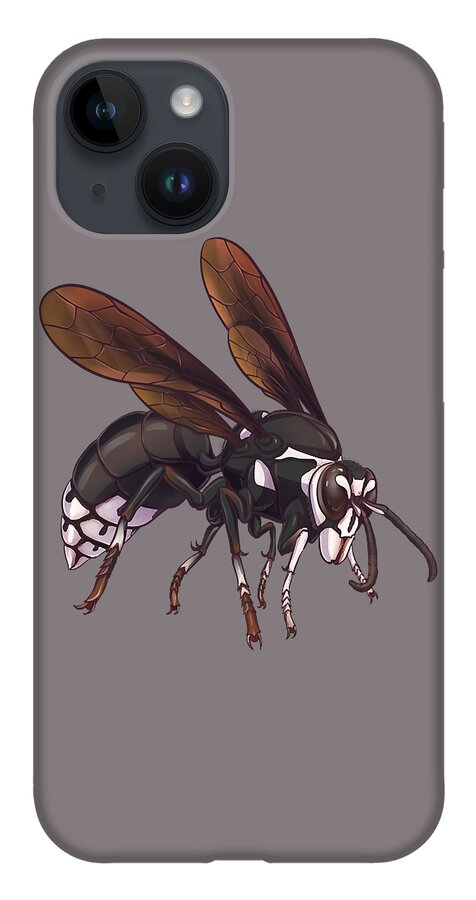This image showcases an AI-generated model of an Apple iPhone encased in a dark gray or mauve phone case. The centerpiece of the phone case is a detailed, illustrated depiction of a large insect, likely a housefly, rendered with a mix of colors including brown, white, purple, black, and shades of gray. The fly's wings exhibit amber hues, while its legs are white with amber tips. The body is predominantly black with a white tail, and the head features a blend of black and white, suggesting a somewhat sinister expression. The insect's design appears to employ a watercolor or marker technique for a somewhat artistic, cartoonish effect rather than a strictly realistic one. The iPhone itself is dark gray slate in color, and there is an opening in the case for the dual lenses of the camera and a flash. The white background gives the impression that this is a professional product image rather than a casual photograph.